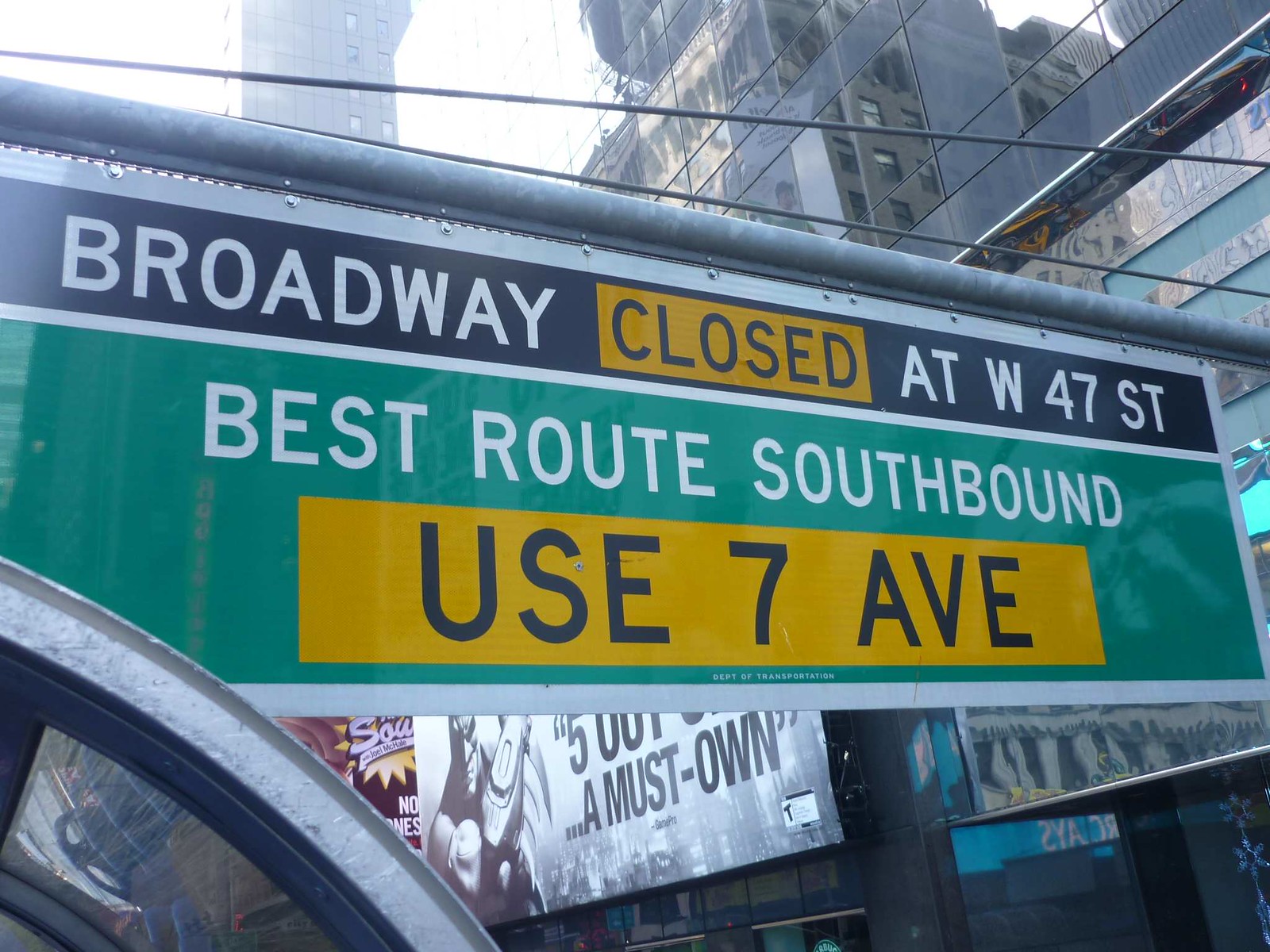This image depicts a street sign in a bustling urban environment, likely New York City, given the tall skyscrapers with mirrored windows in the background. The photograph is a large, rectangular shape and was taken outdoors during the daytime, with a glimpse of bright white sky visible in the upper left-hand corner. The sign itself is rectangular but hangs from a silver or gray metal bar stretching horizontally above it.

The sign is divided into distinct sections with various colors and text. At the top is a thin white strip, beneath which lies a thicker black strip. On the left side of the black strip, in white capital letters, it reads "BROADWAY." In the middle of the black strip is a yellow rectangle with black capital letters stating "CLOSED." Further to the right, still on the black background, it reads "AT WEST 47TH ST" in white capital letters.

Below this section, separated by another thin white line, is a green strip extending horizontally. In white capital letters, the text says "BEST ROUTE SOUTHBOUND." Beneath this, in a yellow or orange rectangle with larger black letters, it advises "USE 7 AVE."

Around the sign, various elements capture the essence of a vibrant city. Wires stretch across the view above the sign, and modern signage adds to the urban landscape. To the lower left of the sign, there's an archway typical of subway entrances, and in the lower right corner, partial advertisements can be seen, including one for a Batman video game. The detailed elements emphasize the dense, busy atmosphere of this major city intersection.